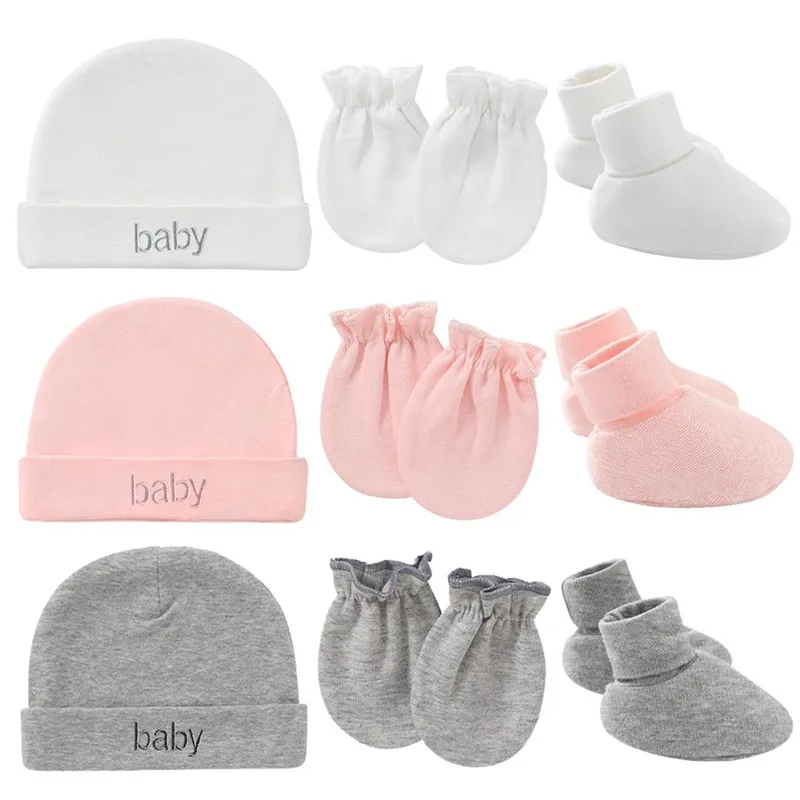This product photograph showcases three sets of baby accessories, meticulously arranged against a pristine white background. Each set consists of a hat, mittens, and booties, organized in three distinct rows. The top row features all-white items, the middle row displays pink items, and the bottom row presents gray items. 

The hats, positioned on the left in each set, are simple beanie-style caps with a folded brim that bears the embroidered word "baby" in the center. To the right of the hats are the mittens, designed with a cinched, elasticized wrist to ensure a snug fit. Furthest right are the booties, which are soft and plush with a narrow cuff at the top to keep them securely in place. Each element in the sets is identical in design, differing only in color, creating a visually harmonious and organized display.